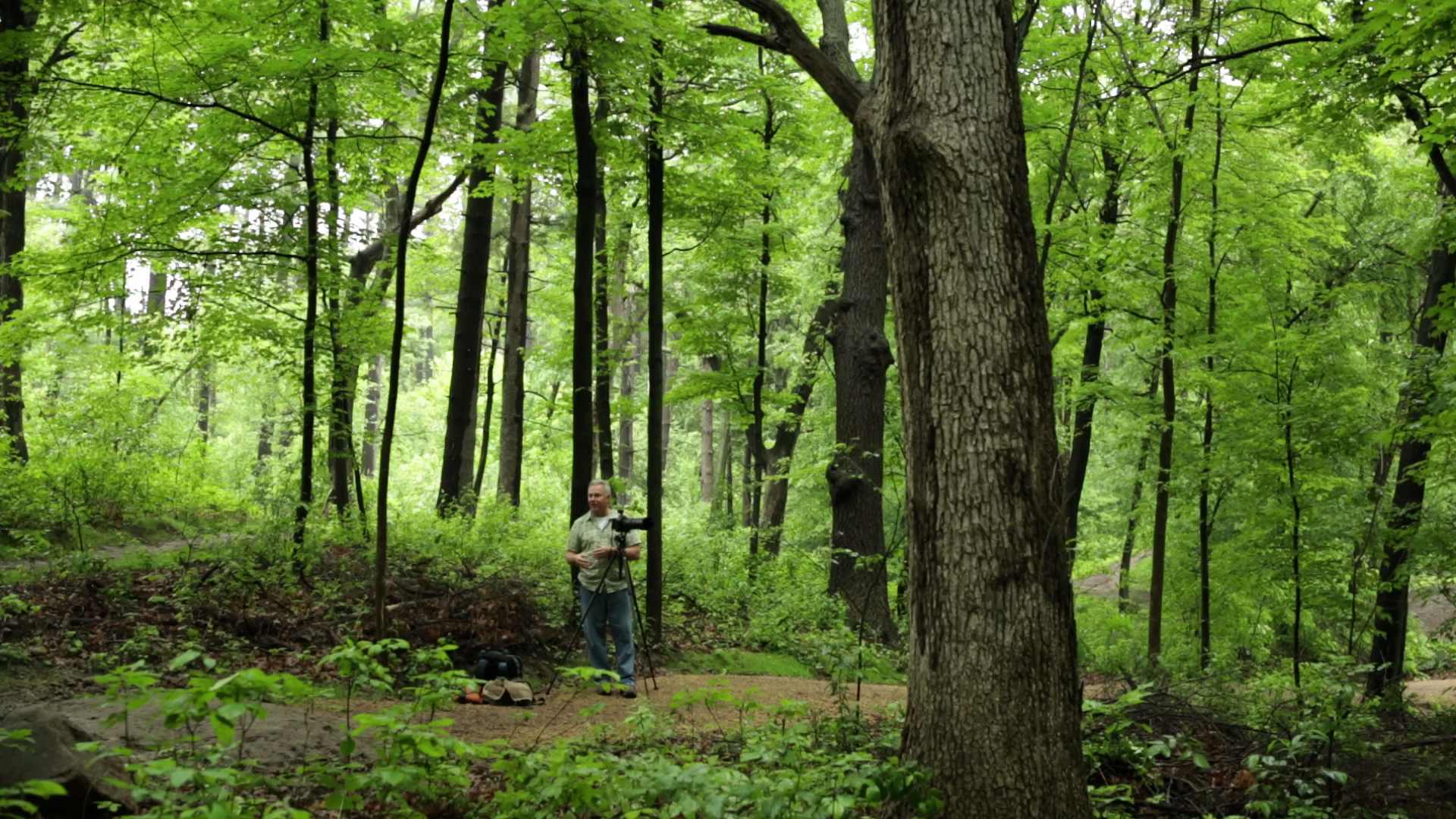In this vibrant color photograph, an older photographer with gray hair stands in the middle of a luscious, green forest, surrounded by dense vegetation and tall trees that are just beginning to bud with fresh green leaves, signifying springtime. The man is centrally positioned on a winding dirt path that snakes off into the distance, with a gentle hill descending from the right-hand corner of the image. He is wearing jeans and a light green, short-sleeved button-up shirt over a white undershirt. A camera mounted on a tripod stands beside him, aimed towards the right, featuring a telephoto lens, potentially indicating it's either a modern or film camera. By his feet, near the bushes and trees, lie several bags of camera equipment. The scene showcases the tranquil yet thriving forest environment where the photographer appears deeply engaged in capturing the natural beauty around him.